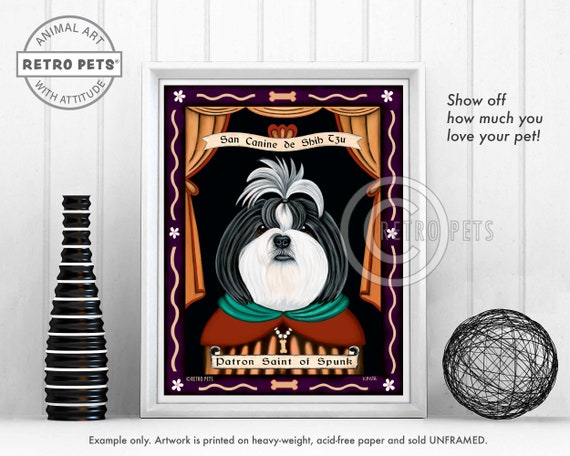The image features a white background with a tile plank pattern. At the bottom of the image, on a white surface, there is text in black that reads "Example only." The artwork showcased is printed on heavy-weight, acid-free paper and is sold unframed, as indicated by the label in uppercase letters.

The main focus of the image is a white rectangular picture frame displaying a dog with a coat featuring white, brown, and black fur. The dog is adorned with a green shawl-like guard around its neck, red at the bottom, and a white chain with a dog bone pendant. 

To the right of the picture frame is a black decorative circle, while on the left side, there is a black and white vase with a striped pattern predominantly showcasing the two tones.